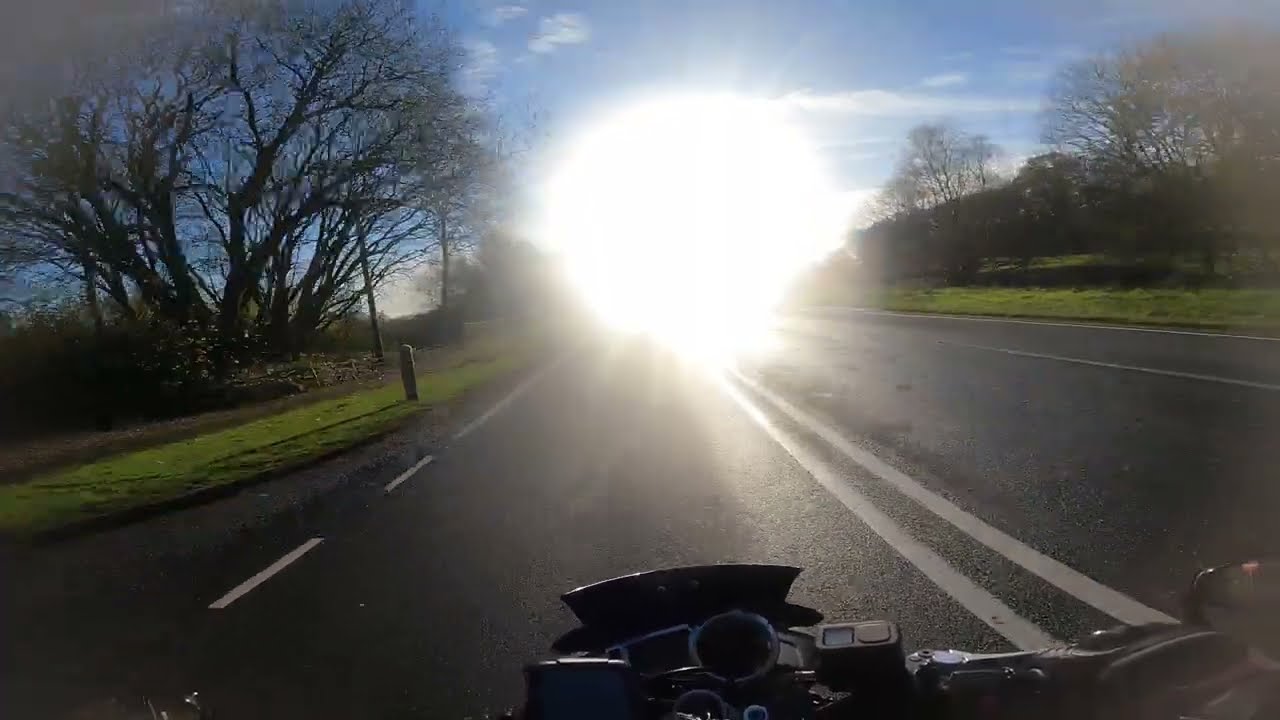The image captures a motorcyclist's perspective as they ride down a black asphalt road during the daytime, with the camera mounted either on the helmet or handlebars. The road features two solid yellow lines dividing its middle and intermittent white lines on the left shoulder; the right shoulder has an unbroken white line that demarcates the pavement from an adjacent bike path. The scene is dominated by a dazzlingly bright, fuzzy white light directly ahead, possibly the low-lying sun, which obscures the distant horizon and creates a high-contrast effect. The sky is blue with wispy, thin clouds scattered across it. On either side of the road, there's green grass and several leafless trees, indicating the season might be late fall or winter. Off to the left, amidst the grass, stands a dark, three-foot pole with a rounded top and a large, multi-stemmed tree trunk with sparse foliage. On the right side, past the bike path, faint stripes mark the continuation of the road, and behind this area, a dark mound, possibly a mountain, can be seen in the background.